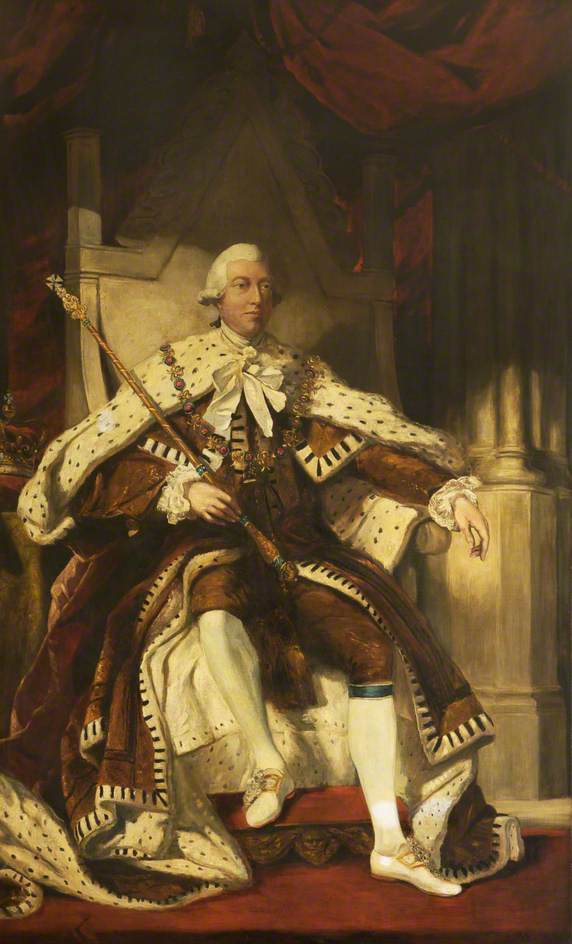This vertical, rectangular painting depicts a self-portrait of a regal figure, likely a king, seated in a throne room. The man, who is of significant importance, is perched on a wooden throne that rises to a tall, triangular point at the back, suggesting his high status. He wears a white, curly powdered wig that curls slightly above his ears, indicating a period style.

The king is adorned in an opulent red outfit resembling velvet, with white shoes and long white socks that reach up to his knees. His pants are tied just below the knee with black ribbons. His red coat, detailed with white and black dotted fur on the collar, cascades over the throne and onto the floor. He's draped in a plush fur cape, distinguished by its brown spots and secured by a large white satin ribbon. His attire includes ruffled sleeves and a brown jeweled necklace that drapes across his shoulders and chest.

In his right hand, he firmly holds a long, wooden staff with brownish-gold accents, while his left hand rests on the throne's armrest. The background of the painting features a darkened upper section that contrasts with the red carpeted floor of the throne room. Flanking him are gray columns, hinting at the grandeur of the setting. The overall color scheme of the image is a blend of reddish, brown, and beige tones, adding to the majestic and regal atmosphere of the portrait.